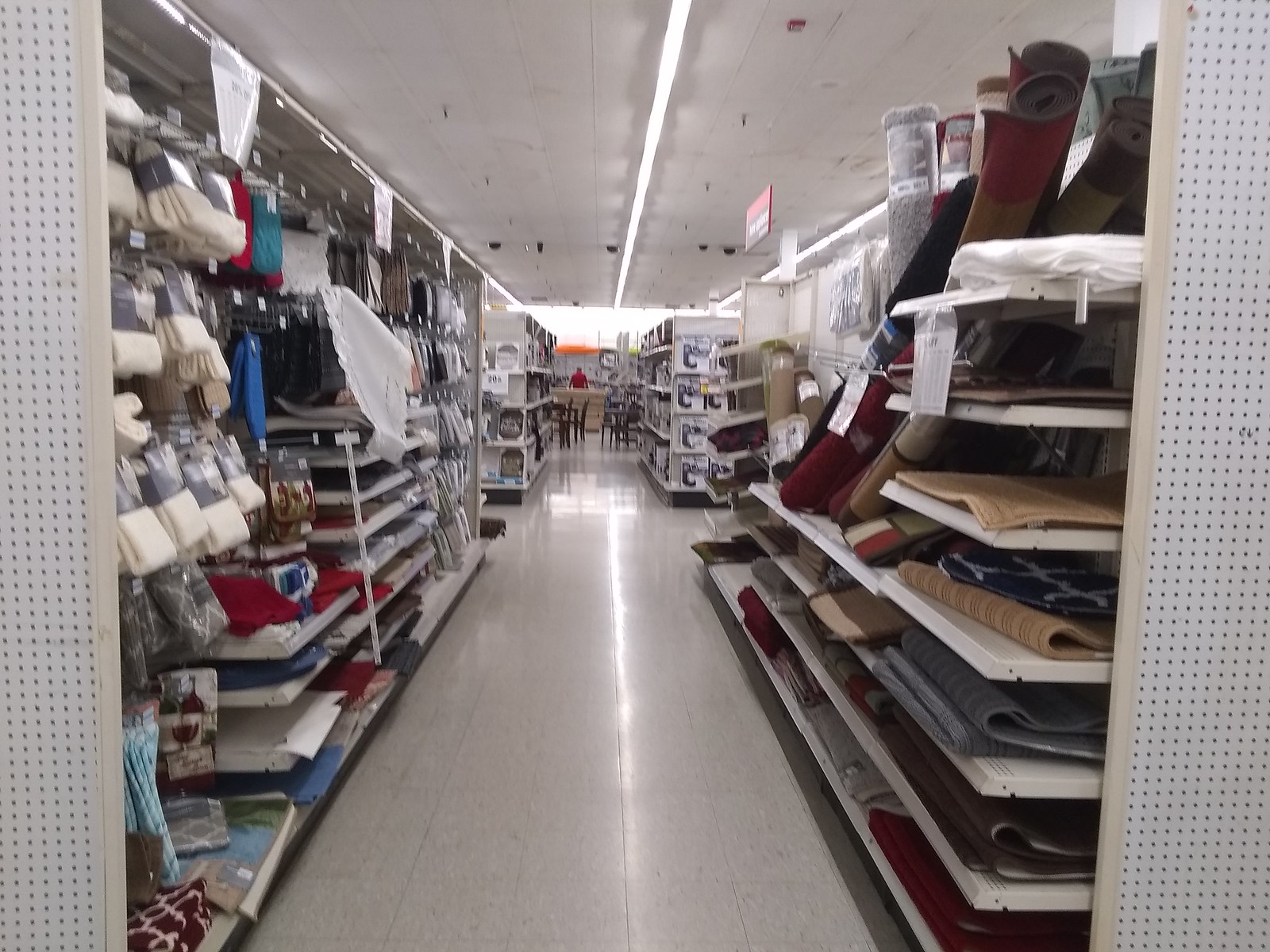This photograph captures the interior aisle of a home goods section within a department store. The scene is framed by white tiled ceilings and a matching tiled floor, emphasizing the orderly layout of the store. On the right side of the aisle, there are seven shelves, each stocked with a variety of small area rugs and doormats. The rugs display a range of colors, from red and brown to blue and white, with some larger rugs rolled up and standing vertically on the top shelf. The foreground features an assortment of doormats piled up in various hues including red, black, dark blue, beige, and pure white.

On the left side, the shelves are filled with an assortment of hand towels or rags and possibly potholders, neatly folded and packaged. The shelving units are adjustable with a grid of holes, allowing flexibility in their configuration. The aisle extends forward, revealing another row of shelves in the distance with a person in a red shirt standing at the far end, under the store’s overhead fluorescent lights. The overall composition conveys the tidy, stocked nature of this home goods section, highlighting the organized and varied selection available.